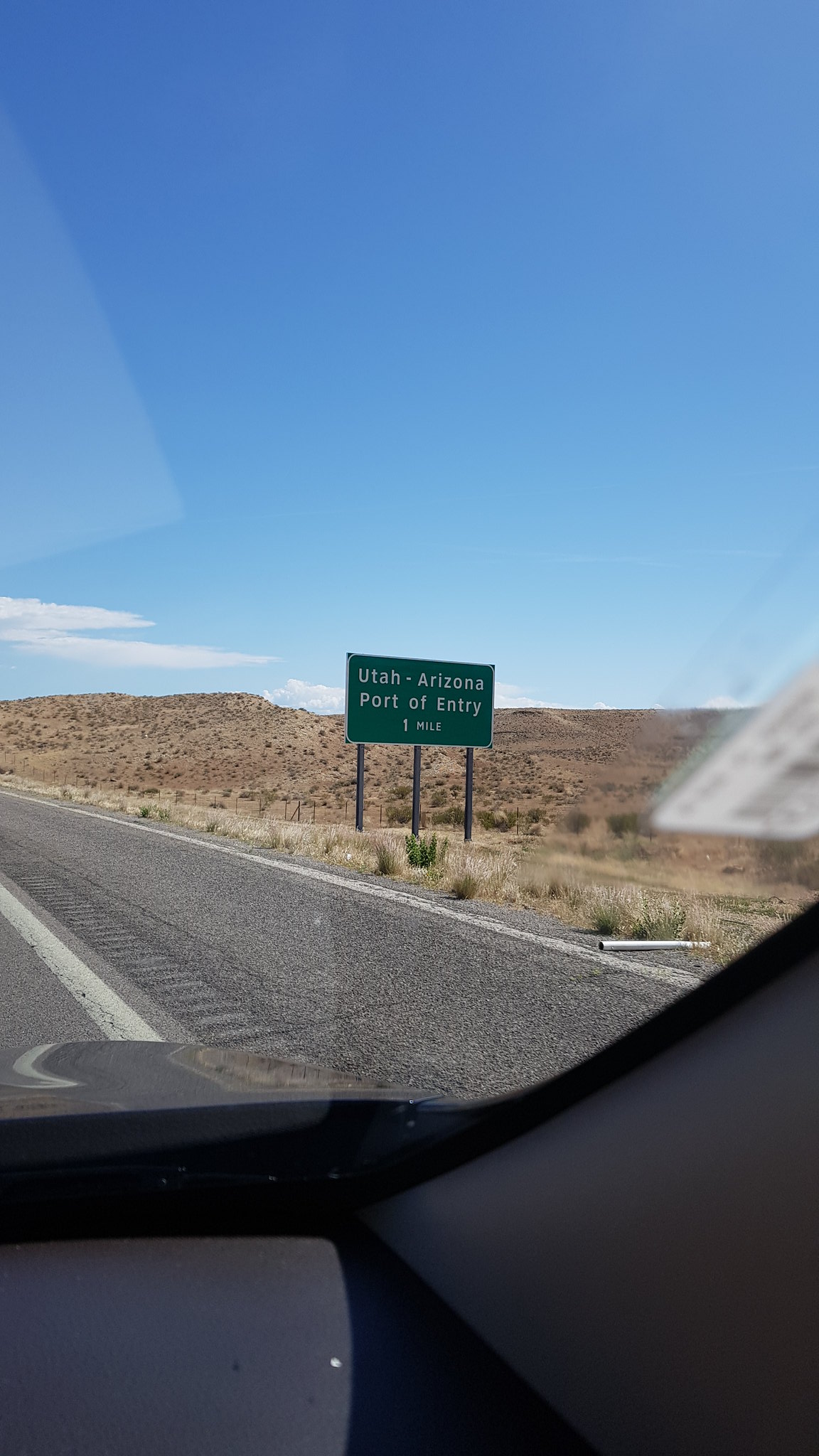Photographed from the passenger seat of a car through the windshield, this image captures a road sign against a stark and barren landscape on a highway. The scene features rolling, hilly terrain with a light brown, dusty ground interspersed with sparse, small green shrubs, emphasizing the arid conditions. Above, the sky is a crisp, clear blue with only a handful of scattered clouds. The rectangular green road sign, supported by three evenly spaced vertical posts, prominently displays white text that reads "Utah-Arizona Port of Entry 1 Mile." The sign and the surrounding environment underscore the dryness and simplicity of the landscape, punctuated by the smooth asphalt of the highway stretching ahead.